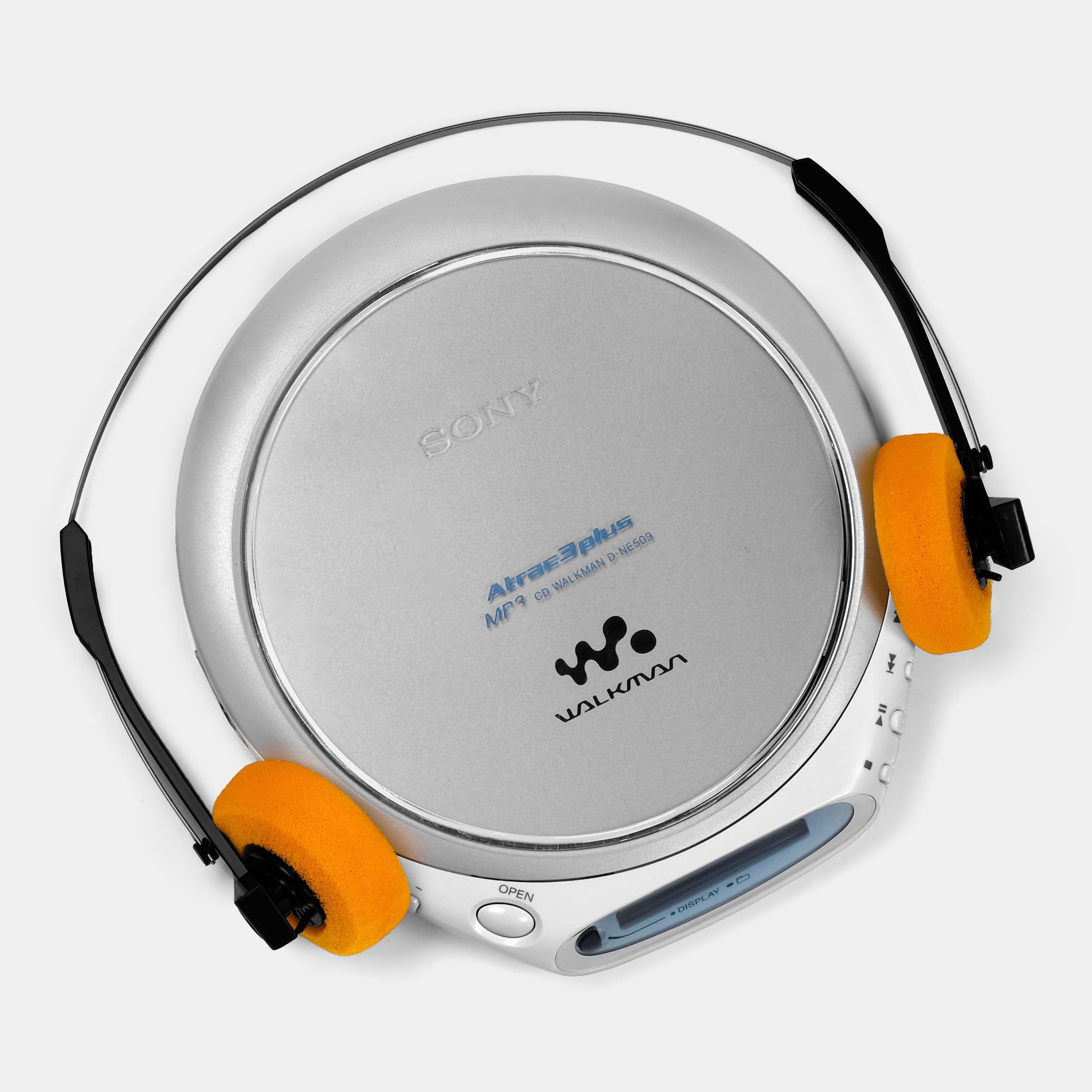This is an overhead image of a vintage Sony CD Walkman from the early 1990s to early 2000s. The Walkman has a distinctive circular silver top with "Sony" branding prominently displayed on it. The model is labeled as an "Ultra 3 Plus MP3 CD Walkman." At the bottom right of the device, there is an open button for accessing the CD compartment, and to the left, there are various playback controls, including play, pause, forward, and stop buttons. The front of the Walkman also features a small oval digital display for indicating track numbers. Resting on top of the Walkman is a pair of thin metal-framed headphones with extended black arms and bright orange foam covering the ear pieces. The photo appears to be taken against an indistinct light-colored background.